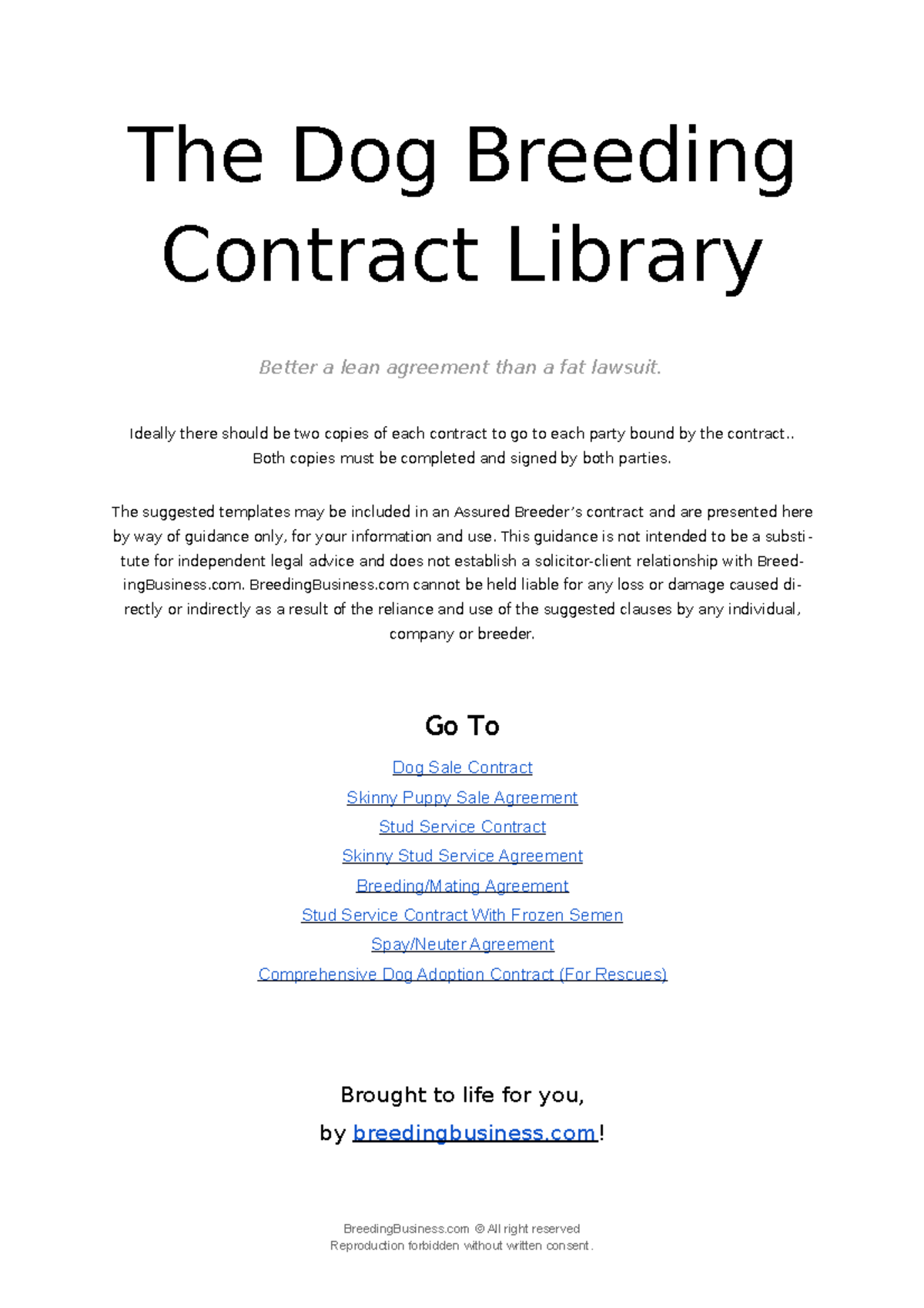This image offers detailed information about a variety of dog breeding contracts. At the top, in bold print, it prominently displays the title "Dog Breeding Contract Library." Below this title, it features the phrase "Better a lien agreement than a fat lawsuit," emphasizing the importance of legally binding agreements in dog breeding.

The text elaborates on the necessity of having two copies of each contract for each party involved, specifying that both copies must be fully completed and signed by all parties. A note indicates that the suggested templates, which are included for breeders' reference, are provided merely as guidelines and not as substitutes for independent legal counsel. It also clarifies that the guidance provided does not create a solicitor-client relationship with the website breedingbusiness.com. Additionally, it mentions that breedingbusiness.com is not liable for any loss or damage resulting from the reliance on or use of these suggested clauses by any individual, company, or breeder.

The image further organizes the information into several sections, listing specific types of contracts available. These include:
- Dog Sale Contract
- Puppy Sale Agreement
- Stud Service Contract
- Stud Service Agreement
- Breeding Mailing Agreement
- Stud Service Contract with Frozen Semen
- Spay/Neuter Agreement
- Comprehensive Dog Adoption Contract for Rescues

At the bottom, the text credits breedingbusiness.com as the source of this information, indicating that they have brought this library to life for the users' benefit.